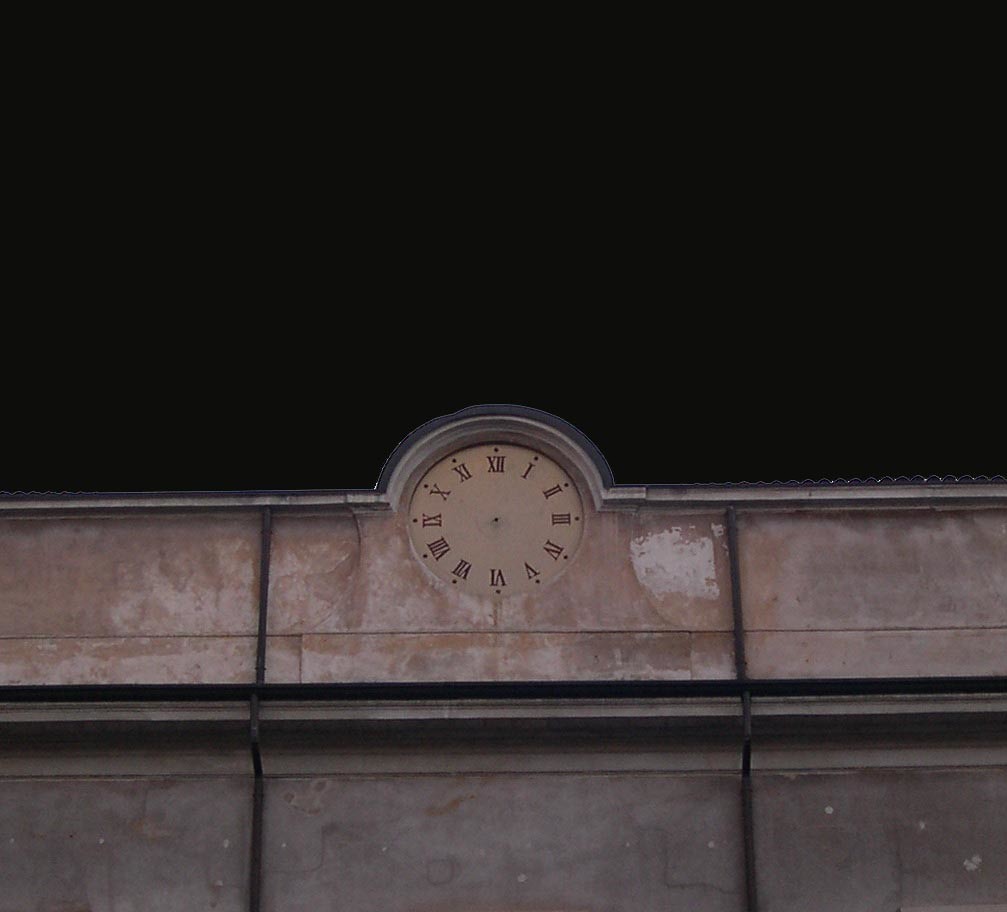The image features a nighttime view of a clock mounted atop a building. The sky behind the structure is a solid, impenetrable black, emphasizing the silhouette and details of the building. The building itself exudes a certain elegance, with its facade transitioning through various shades of rose and gray. The upper left and central sections boast a pale rose-gray hue, while the right side shifts to a slightly darker gray. Below this, a light gray section adds contrast.

The roofline of the building is straight, except for a distinctive, semi-circular projection that houses the clock. This clock is a circular centerpiece with a background of pale parchment gold, giving it a subtle yet dignified appearance. The clock face is adorned with Roman numerals, with the 'XII' at the top, followed sequentially by the numerals marking each hour down to 'XI'. A small circle at the center marks where the clock hands should be, although they seem to be missing, possibly having fallen off.

Adding to the architectural detail, the rose-gray section of the building is flanked by metal gutters above and below and features multiple vertical metal brackets that appear to support or embellish the structure.